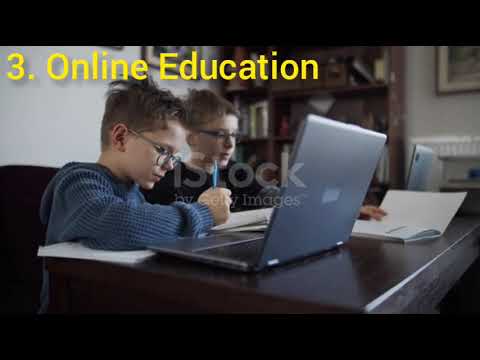This image captures two young boys, who appear to be identical twins, sitting at an adult-sized desk engrossed in their schoolwork for an online education session. Both boys are wearing glasses. The boy on the left, dressed in a black sweatshirt, is focused on an open book in front of him, while the boy on the right, clad in a blue hooded sweater, is writing on a pad of paper with a blue pen, positioned next to an open laptop. A secondary laptop is also visible, suggesting a shared workspace. The setting appears to be indoors, possibly a study or home office, with a bookshelf in the background adding to the academic atmosphere. Text in the upper left corner of the image reads "3. Online Education," and a watermark in the center states "iStock by Gottlieb Images." The overall scene suggests a diligent and organized homeschool environment.